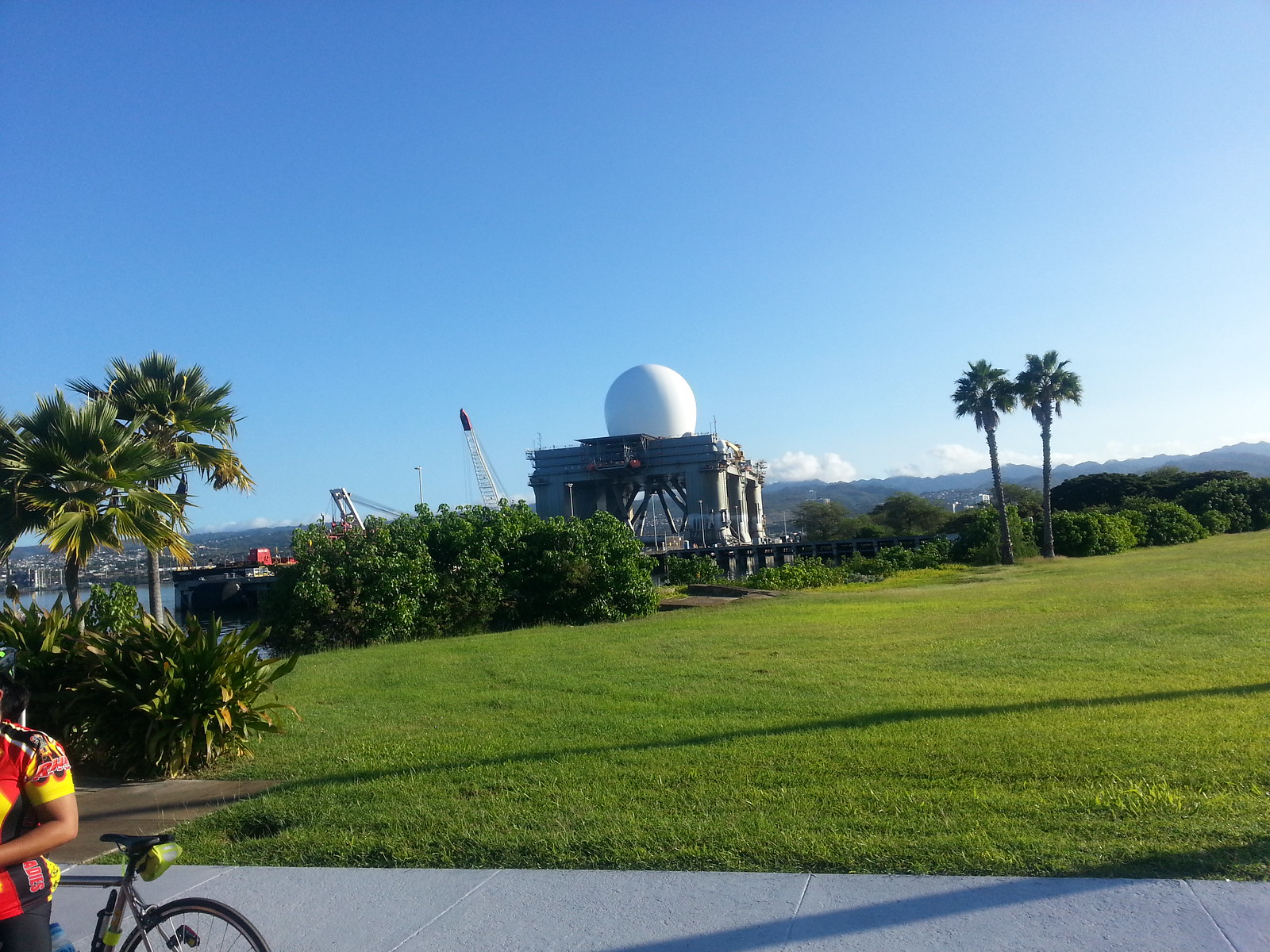In this vibrant daytime outdoor image, a sidewalk stretches across the bottom, leading to a lush, expansive green lawn surrounded by several bushes and at least four or five tall palm trees. In the lower left-hand corner, a person with deep tan skin is standing beside a bicycle, clad in striking red, yellow, and black attire that might be a uniform. The background features a massive, unfinished structure resembling a drilling or oil platform with six gray, metallic legs and a prominent white dome atop it, transitioning in color from white to blue. Two cranes loom in the distant background to the left of the platform. Beyond the platform, there's a body of water, possibly part of an ocean, lake, or river. The sky above transitions from darker hues on the left to lighter shades on the right, enhancing the scene's vividness and depth.